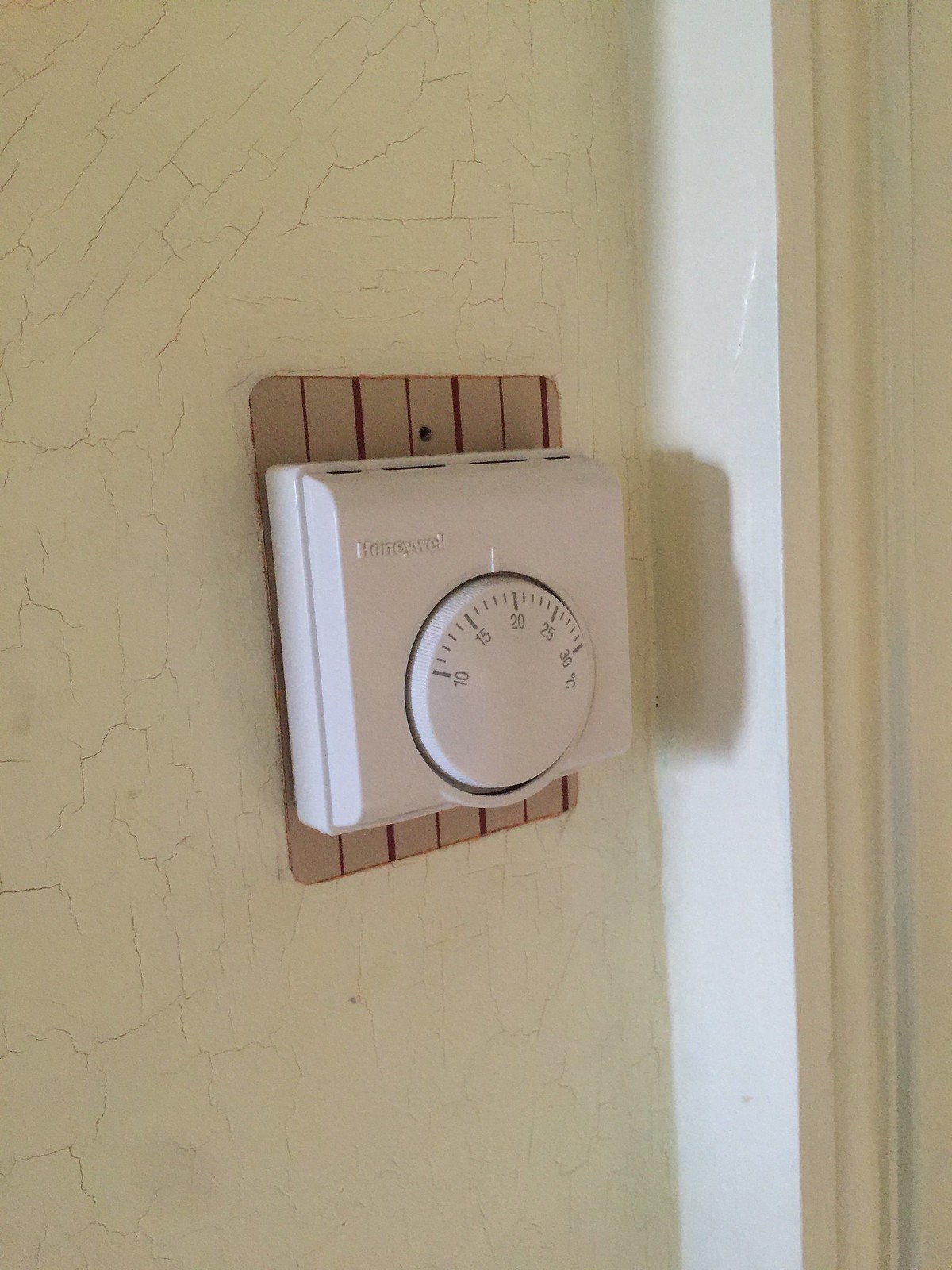This image features a non-digital, all-white thermostat primarily marked in Celsius, manufactured by an unspecified company. The thermostat is affixed to a slightly detached backplate, which notably has a striped pattern. The central dial, which dominates about half of the device's surface area, is set to 20 degrees Celsius and is recessed into the bottom part of the thermostat. 

Above the dial, vents allow for airflow regulation. The wall to which the thermostat is attached is visibly cracked, suggesting potential age or wear, and leads into a somewhat indistinct, softly rounded corner. The lighting in the scene originates from the left side, casting shadows to the right and giving a clear indication of the direction of illumination. The photograph is angled from the left, capturing the thermostat, backplate, and the adjacent wall corner cohesively.